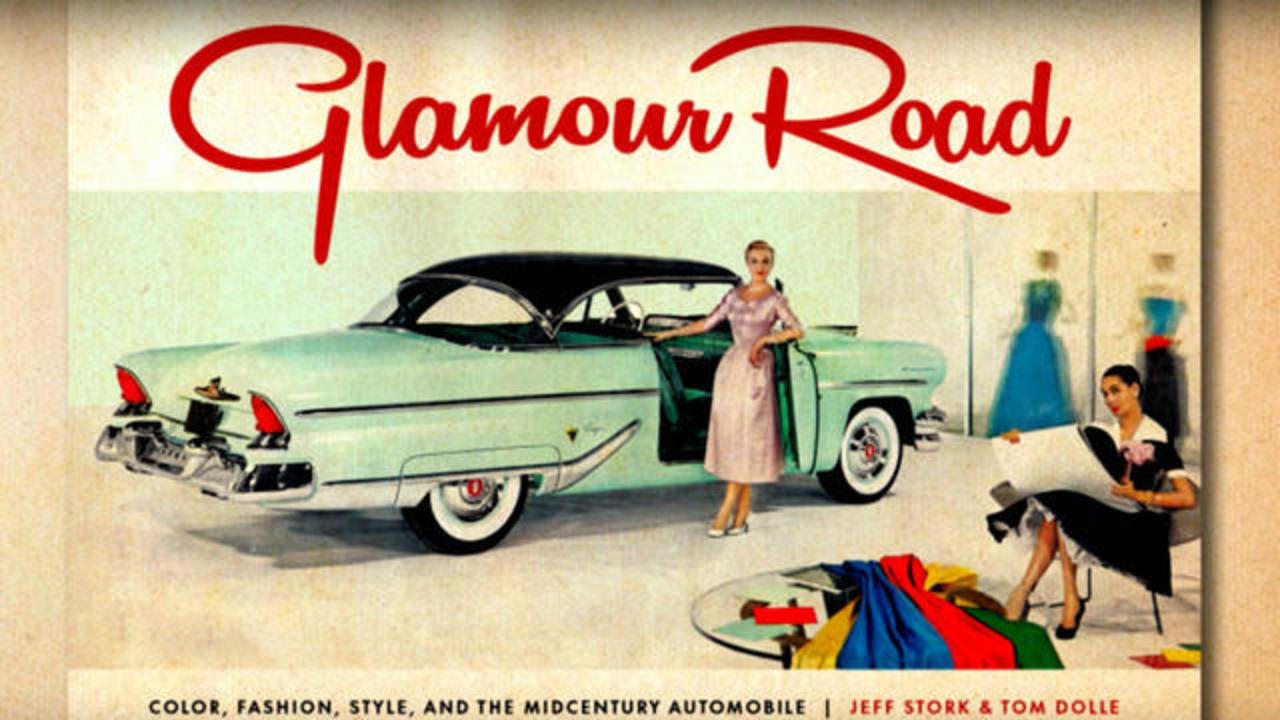This image is an old-styled advertisement reminiscent of the 1950s, with a nostalgic, slightly stained, and time-worn look. At the top, in bold red cursive font, it reads "Glamour Road." Centrally featured is a light turquoise car with a distinct black hood. The car's front passenger side door is open, and a woman, donned in a 1950s style pink dress that reaches a few inches above her ankles and has three-quarter length sleeves, leans against the door. The car's tires are whitewashed with red detailing in their centers. Toward the bottom, the advertisement states, "Color Fashion Style and the Mid-Century Automobile," followed by the names Jeff Stork and Tom Dole. On the right side of the image, there are additional details, including another woman in a black dress sitting and examining various colored fabrics. The scene appears like a photorealistic painting, depicting an indoor showroom filled with mid-century charm.